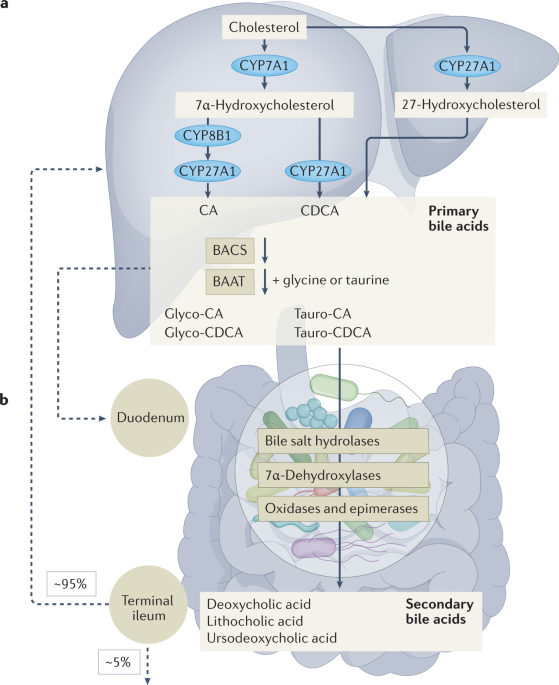The image is a detailed computer-generated diagram illustrating the biochemical processes within the human digestive system, focusing particularly on bile and cholesterol metabolism. Set against a white background with gray bubbles and dotted lines, the graphic includes a schematic representation of the stomach and intestines. Key components in the diagram are labeled with medical and biochemical terms.

At the top, the word "cholesterol" is connected via arrows to various enzymes such as CYP27A1, CYP7A1, CYP8B1, and CYP27A1. These enzymes link to specific compounds like 27-hydroxycholesterol and 7-alpha-hydroxycholesterol, forming part of the metabolic pathway.

Primary bile acids are highlighted in a square, including compounds like CA (cholic acid) and CDCA (chenodeoxycholic acid), which are further modified into glyco-CA and glyco-CDCA through reactions involving glycine or taurine. The enzymes BACS and BAAT are noted in this process.

The digestive organs depicted show additional annotations: "bile salt hydrolysis," "7-alpha-dehydroxylases," "oxidases," and "epimerases," with a dotted arrow leading from the primary bile acids to the intestines. Specific locations within the digestive tract, such as the "duodenum" and "terminal ileum," are circumscribed with arrows illustrating the movement and reabsorption of bile salts, where 95% are reabsorbed back to the stomach and 5% are excreted.

Finally, secondary bile acids—deoxycholic acid, litocholic acid, and ursodeoxycholic acid—are depicted at the bottom of the graphic, underscoring the comprehensive portrayal of bile metabolism in the digestive system.